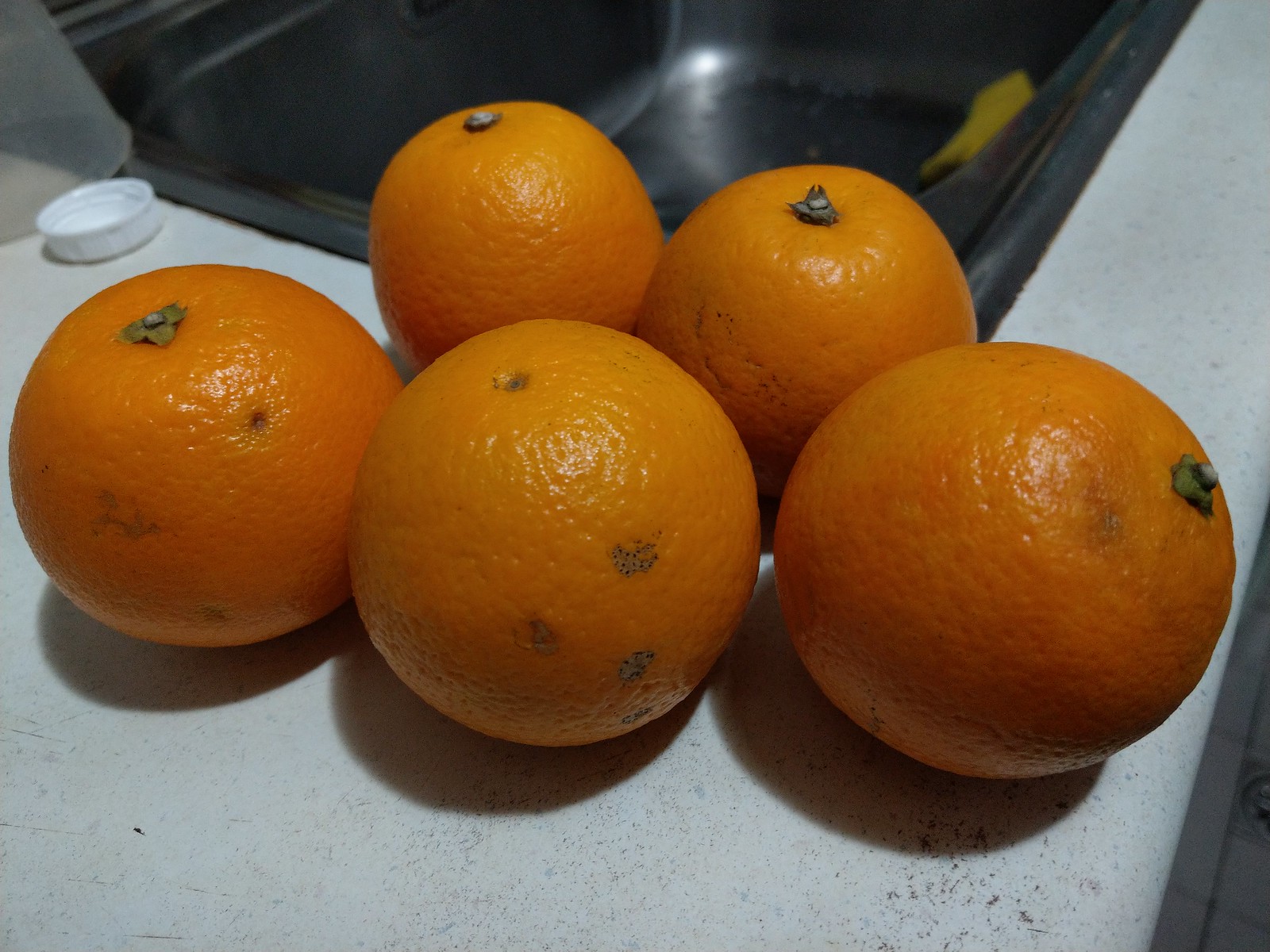The photograph, taken in landscape orientation and slightly out of focus and dark, captures a close-up of five ripe oranges arranged on a speckled white kitchen countertop. The oranges are positioned with three larger ones in a row at the front and two slightly smaller ones behind. A source of light from the upper right casts distinct shadows from the front oranges onto the countertop. The countertop itself is white with tiny bronzy-brown and larger grey-black speckles, especially prominent in the right foreground. Behind the oranges is a black sink, partly visible and slightly cut off at the top of the image. A white, upturned bottle cap sits to the left behind the oranges, near the hem of a kitchen curtain. There is noticeable grime between the sink and the countertop, indicating a need for re-grouting. The oranges, while vividly orange, are slightly dirty, with flakes of dirt visible beneath and adhering to one of them. In the sink, there appears to be another object which is either orange or yellow. The front orange also shows a bit of browning. The front edge of the countertop is visible in the bottom right corner, extending out of the frame. The image ties together the kitchen elements and the presentation of the oranges, capturing a homely, everyday scene.